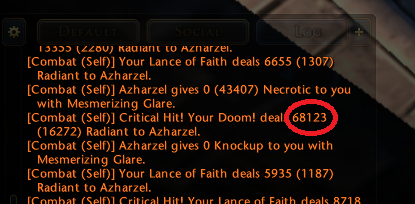This image features a screenshot of a transparent overlay from a video game, showcasing a combat log. The prominent colors include black, orange, and pink. The log, written in orange font against the black background, details a series of combat interactions. The repeated phrases "combat self" are visible throughout, indicating various actions and damage calculations. Specifically, it outlines the damage dealt by "your lance of faith," which ranges from 6655 to 1307 radiant damage to an entity named Azarhal. Azarhal, in turn, inflicts 43407 necrotic damage with a mesmerizing glare. Notably, there is a critical hit by "your doom" dealing 68123 radiant damage, circled in red for emphasis, followed by a subsequent hit of 16272 radiant damage. This detailed combat log also highlights the critical hit and the repeated exchange of damage between the player and Azarhal.